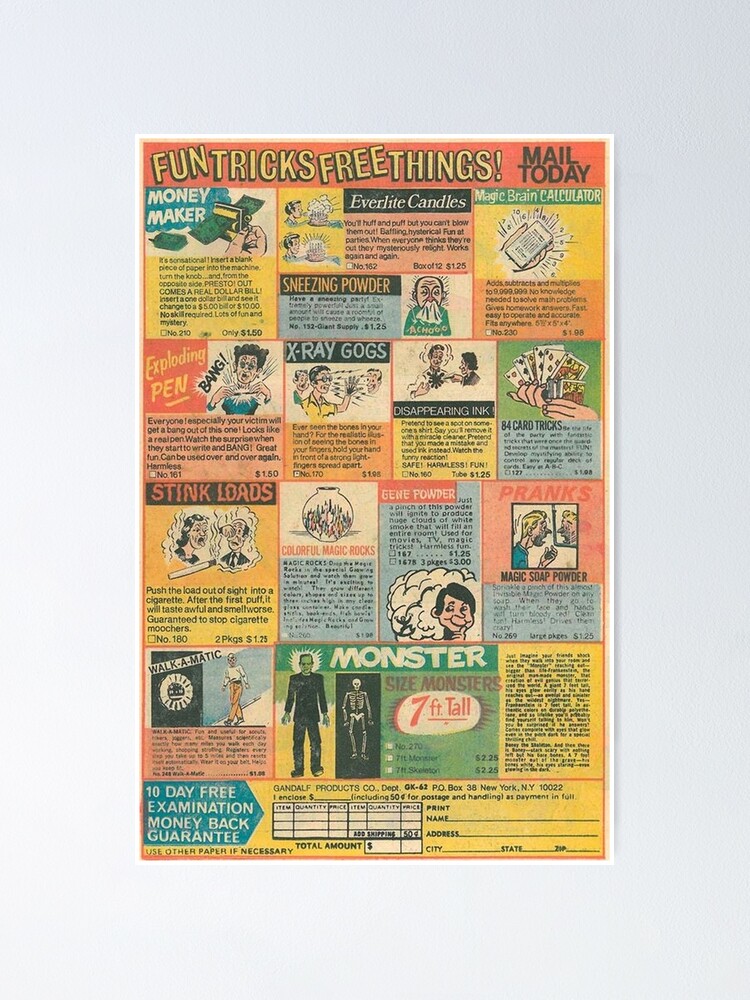The image depicts an old-style advertisement page reminiscent of those found in vintage comic books, likely from the 1960s based on its design and condition. It's filled with colorful cartoon illustrations of various gag gifts and prank items, including x-ray glasses, sneezing powder, pretend money, ever-light candles that can't be blown out, a magic brain calculator, and a card trick book. The page is sectioned into small squares with each product described in detail, accompanied by prices. The top of the page features a bold, eye-catching yellow text within an orange section that reads, "Fun Tricks, Free Things, Mail Today." The background is a muted off-white, displaying wear and tear typical of aged paper. At the bottom, there's a fill-out form for ordering the items, promising a "10-day free examination" with a "money-back guarantee." The whole page sits against a solid gray backdrop, which dominates the photo, emphasizing the vintage advertisement's colorful array.